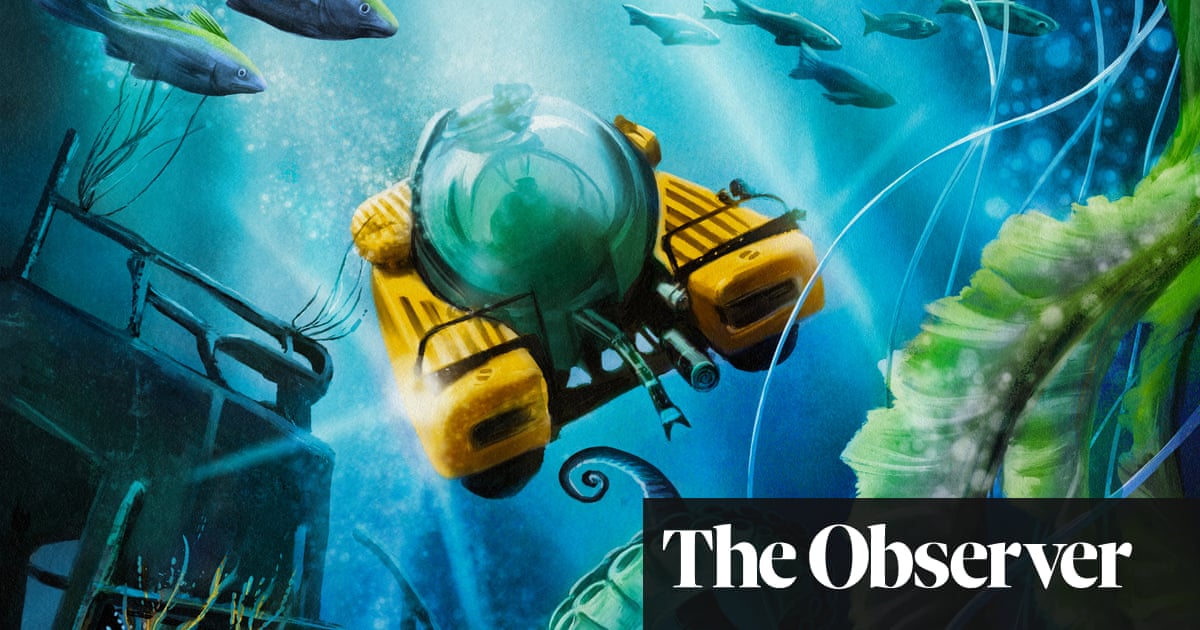This is a detailed illustration, possibly a computer-generated image or a painting, depicting an underwater exploration scene. At the bottom right-hand corner of this rectangular image, which measures approximately six inches wide and three inches high, there's a horizontal black rectangle with the words "The Observer" in white text, suggesting it might be from a publication like a newspaper or magazine. The scene highlights a yellow underwater vessel, with two elongated yellow tubes, or engines, on either side. The focal point of the vessel is a large, clear, globe-shaped windshield which appears slightly bluish-green, through which a pilot can be seen. The vessel is equipped with lights, a grappling bar at its center, and a long metal hook extending from its front. Surrounding the vessel, the underwater environment is detailed with blue water, bubbles, various fish, and tall green seaweed on the right. To the lower left of the image, remnants of a shipwreck can be seen, adding to the exploration theme. Additionally, a tentacle, likely from a sea creature such as a squid, extends upwards towards the vessel, complete with visible suction cups, adding an element of underwater mystery and adventure.